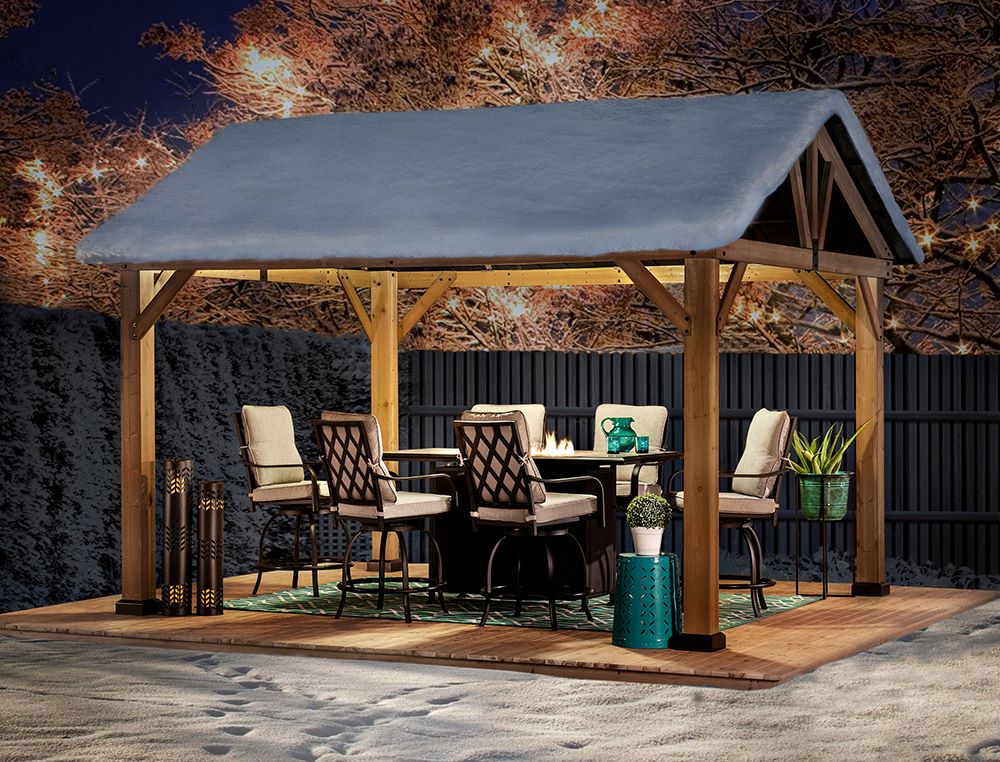The image depicts a cozy outdoor patio or gazebo situated in a backyard. The open structure is supported by wooden beams and topped with a gray roof. Intriguing is the fact that both the roof and surrounding ground appear to be covered in snow, suggesting either a recent snowfall or an intentional decorative touch to evoke a winter atmosphere. 

The patio is enclosed on one side by a brown fence, which is partly adorned with greenery, adding a touch of nature to the otherwise wintry scene. Beneath the shelter, a glass-top dining table is surrounded by six chairs. The chairs are designed with white cushions and feature intricate black and white crisscross patterns on their backrests, enhancing the overall elegant aesthetic.

On the table, various items are meticulously arranged, including a green water pitcher paired with a matching glass, and possibly salt and pepper shakers. A plant in a holder is placed to the right, while another plant sits on a green block within a white planter, adding layers of texture and greenery to the space. The center of the seating area is defined by a green carpet, bordered by a surface that could be brown and beige wood or cement.

The patio is further warmed by the presence of two brown and gold heaters on the left, ensuring comfort in the cold setting. Overhanging lights are strung between the surrounding brown trees, which indicate a fall or early winter environment, casting a gentle glow and adding to the inviting ambiance of this winter-themed outdoor retreat.